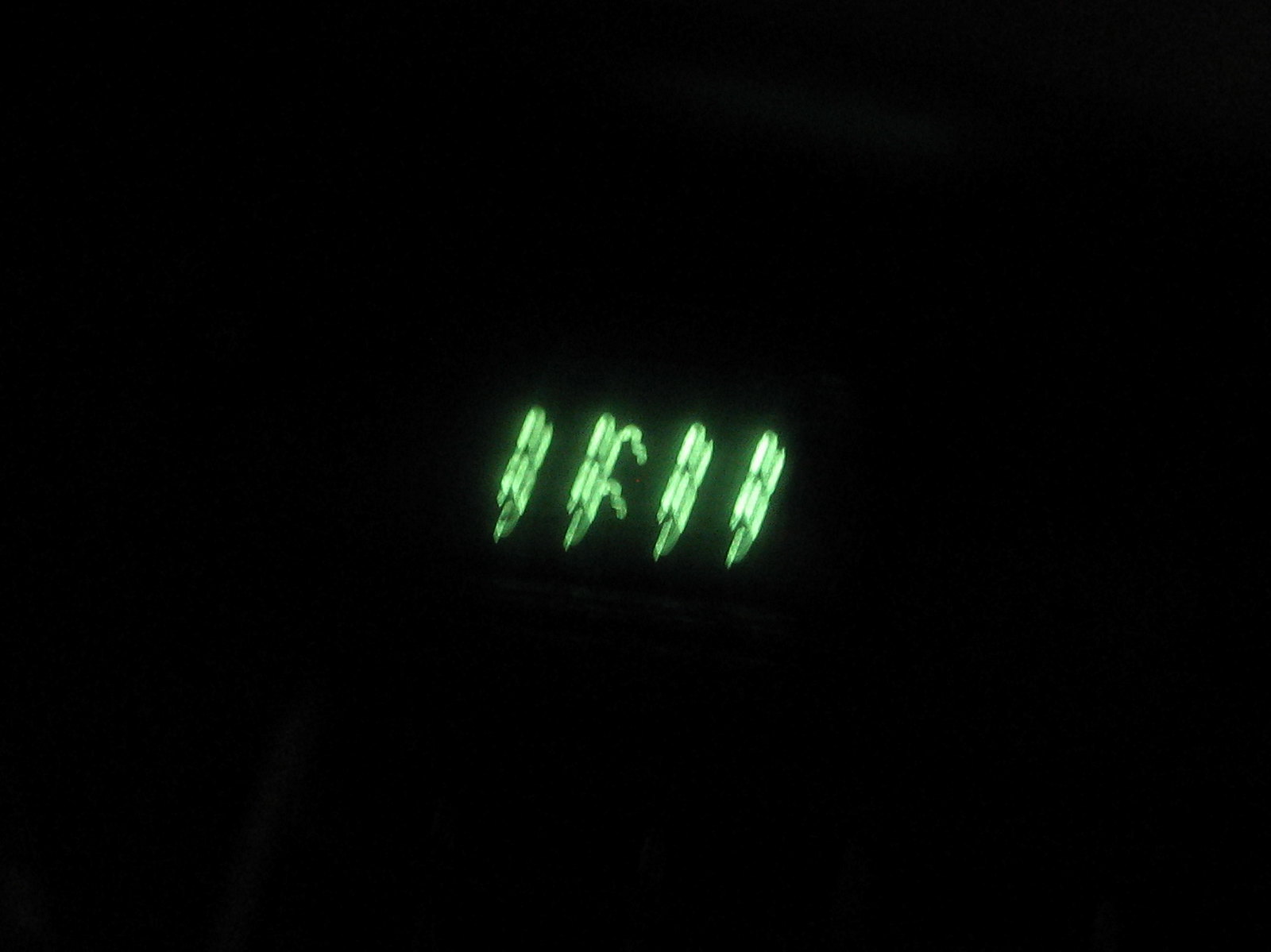This photograph showcases a striking green neon installation set against a pitch-black background. The neon lines extend diagonally from the lower left to the upper right, almost reaching a vertical orientation with a slight tilt. The composition features four distinct neon lines; three are identical in shape, while the second neon line from the left uniquely diverges with two angled segments jutting off to the right, resembling the delicate antennae of an insect. The sharp contrast between the vivid green glow and the deep black background accentuates the intricate details and geometric abstraction of the neon design.